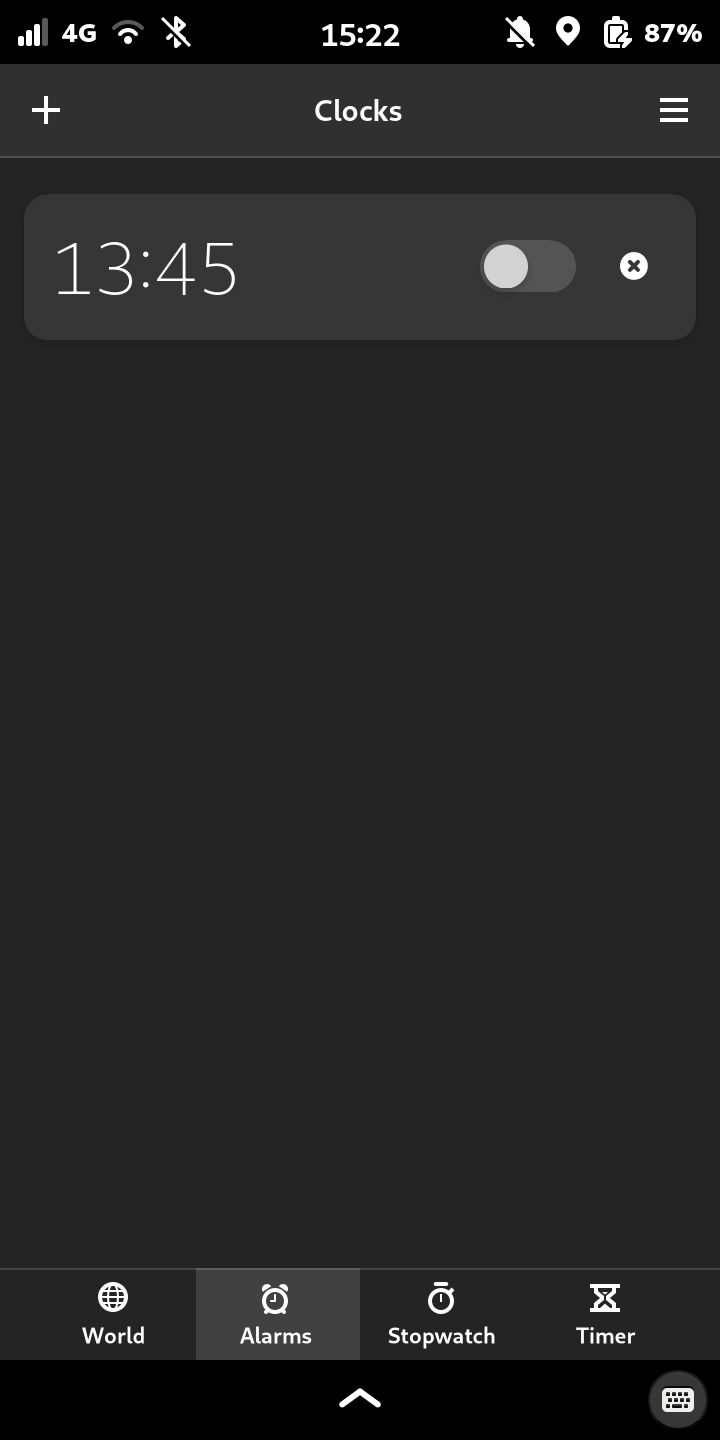The image displays a smartphone screen with Bluetooth enabled and the time indicated as 13:22. A crossed-out bell icon signifies that notifications are silenced. The battery is critically low at 7%. Alongside, the screen shows a clock section within a handbook menu, now displaying the time as 13:45. The current screen section is labeled "Sectors Alarms," illustrated by a classic alarm clock icon with two bells on top. Other sections include "World" and "Stopwatch," indicated by a grayed-out background and navigational elements. There is an up arrow at the top of the screen, and the bottom right corner appears shaded. The interface also contains a virtual keyboard, and multiple icons and menus are cluttered throughout the bottom of the screen, suggesting an elaborate and detailed clock application.